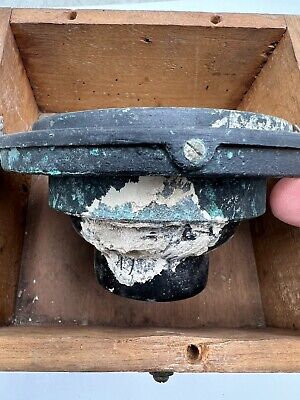This detailed color photograph depicts an ancient-looking, rusted metal valve device situated partially inside an old, lid-less wooden box with drilled holes along its top edges. The rectangular-shaped image showcases the heavily corroded valve, consisting of multiple disc-shaped tiers that decrease in size from bottom to top. The valve, originally dark blue but almost black now, reveals patches of chipped paint, exposing extensive rust and a thick layer of white calcium buildup. A flathead screw is visible on one end with remnants of green corrosion, suggesting severe wear, possibly likened to acid corrosion as seen from an old battery. The scene includes a fingertip—likely the middle finger of a person—on the right side of the image, gently holding up the deteriorating device. The wooden box rests on a flat white surface and houses some dust and corrosion flakes, especially gathered on the left side at the bottom, emphasizing the artifact's aged and decrepit state.